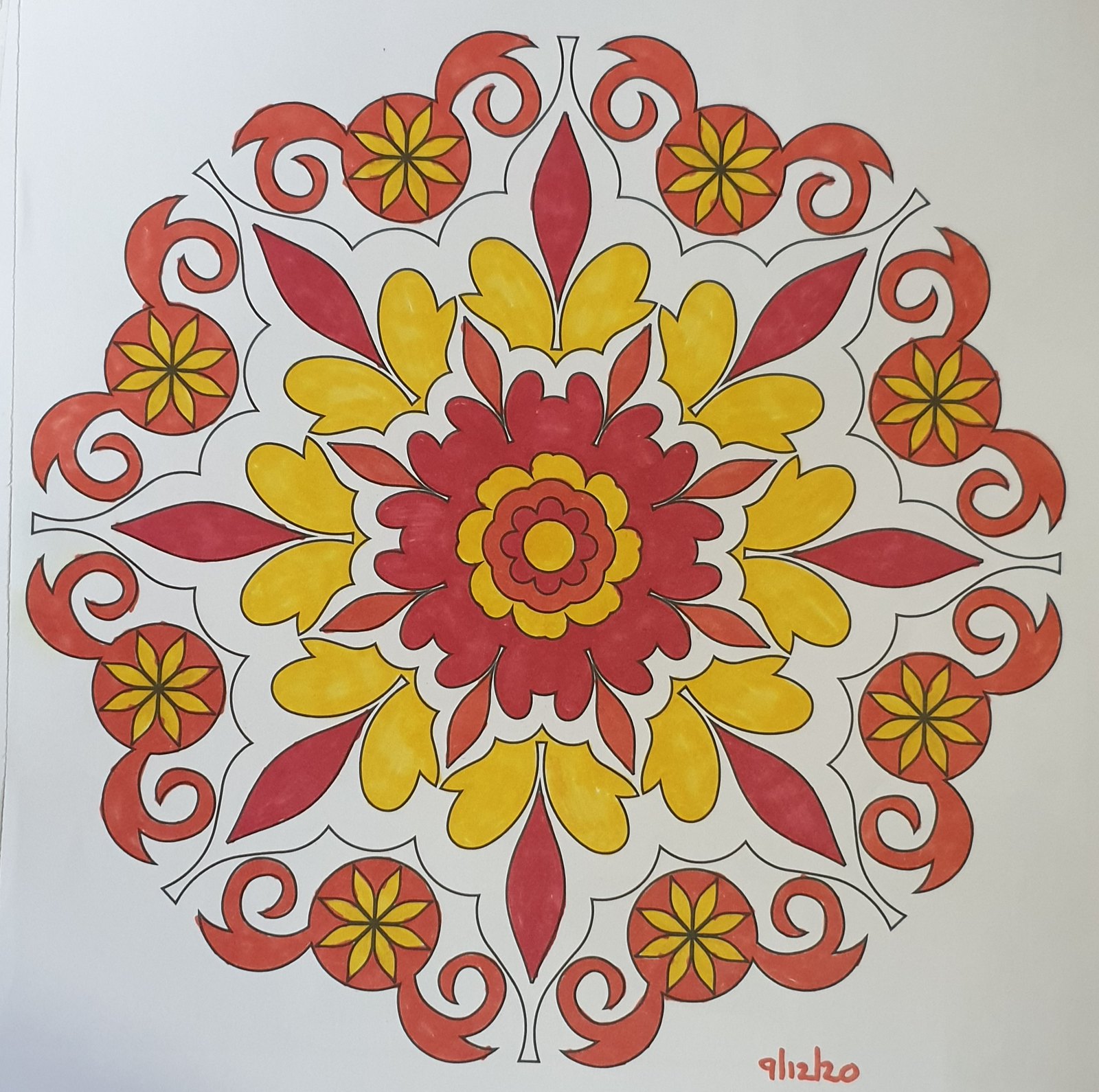This vibrant artwork is a hand-colored mandala, featuring intricate floral and botanical designs, rendered with markers. The drawing employs a black ink outline, meticulously applied with a thin line pen, to define its detailed patterns. The piece is set against a pristine, solid white background. Positioned at the bottom right corner, an orange marker note reads "9/12/20," likely indicating the date of completion. At the heart of the mandala, a central flower blooms, surrounded by a harmonious arrangement of leaves and additional flower-like forms, layered outward in a rhythmic progression. The coloring, dominated by warm hues of orange, yellow, and red, adds a dynamic and radiant quality to the piece, enhancing the depth and complexity of the design.